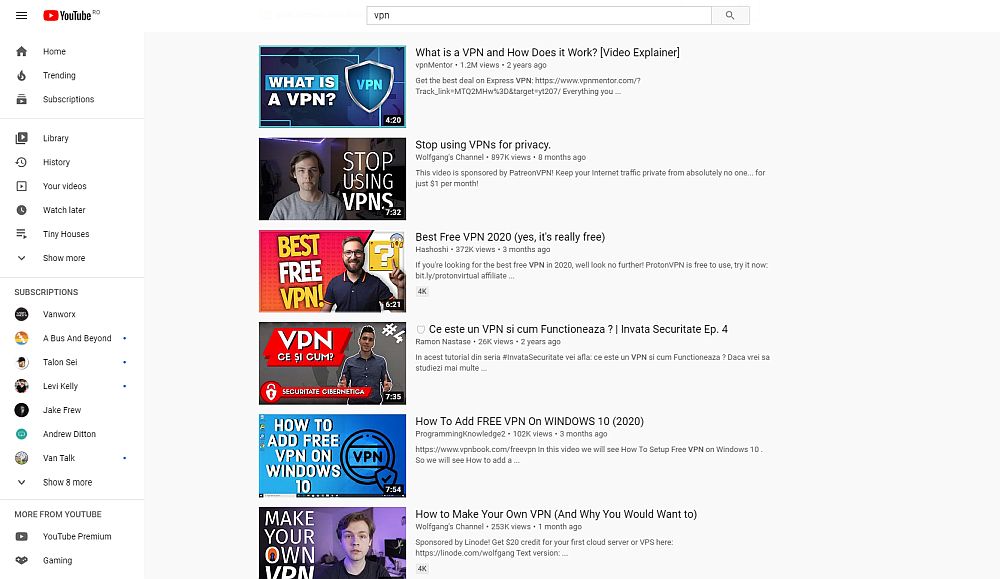The image showcases a YouTube interface with "VPN" entered in the search bar. 

In the top left corner, the familiar YouTube logo is prominently displayed next to the word "YouTube." Below this, the left sidebar features a series of categories, each accompanied by an icon. These categories include: 

- Home
- Trending
- Subscriptions
- Library
- History
- Your videos
- Watch later
- Tiny houses
- Show more

Under the "Show more" option, additional categories are listed, such as:

- Subscriptions
- Van Works
- A Bus and Beyond
- Talon Say
- Levi Kelly
- Jake Frew
- Andrew Ditton
- Van Talk
- Show eight more

Below these, there's another section titled "More from YouTube," featuring options like "YouTube Premium" and "Gaming."

On the right side of the screen, search results for "VPN" are displayed, each accompanied by a thumbnail image. The search results include:

1. "What is a VPN and How Does it Work" by Video Explainer.
2. "Stop Using VPNs for Privacy."
3. "Best Free VPN 2020 - Yes, It's Really Free."
4. A result in French.
5. "How to Add Free VPN on Windows 10 2020."
6. "How to Make Your Own VPN and Why You Would Want To."